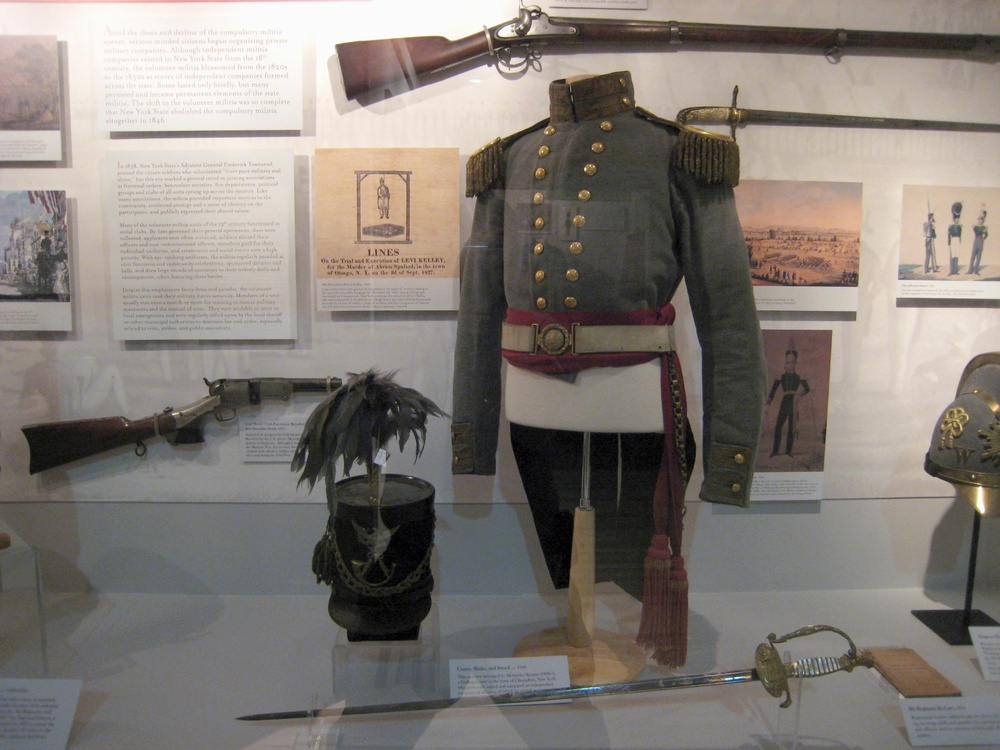The image depicts a detailed Civil War museum display set behind a glass case. Central to the display is a complete soldier's uniform, positioned on a headless mannequin. The uniform features a gray coat adorned with two rows of gold buttons along the lapels, intricate shoulder epaulets with hanging strings, and a tight collar. A vibrant red sash and a decorative white belt encircle the waist of the coat, which pairs with dark trousers. To the left of the uniform is a tall black cylindrical hat, embellished with a metal chain and a distinguished black feather, resting on a stand.

Arrayed around the uniform are various weapons, including two long rifles and two swords, one of which lies on the floor in front of the mannequin. The display is meticulously organized, with white placards providing informational text about each item. The white wall in the background hosts numerous black-and-white photographs of men in similar military attire along with accompanying descriptions, enhancing the historical narrative presented. The entire scene is encased in glass, reflecting light and underscoring the careful preservation of these historical artifacts.